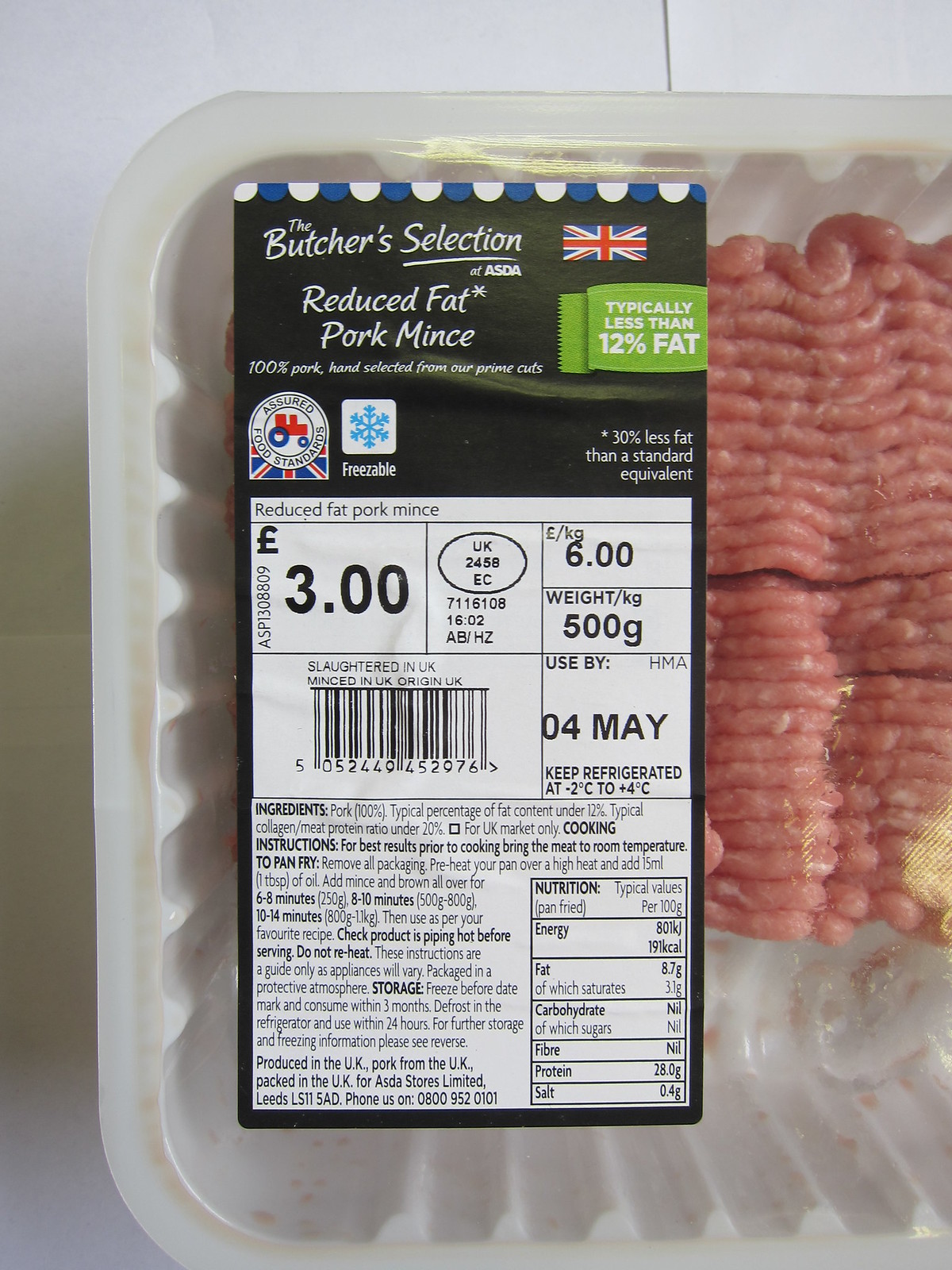This detailed, close-up image taken indoors depicts a 500-gram package of ASDA's "Butcher Selection" pork mince. The package sits on a well-lit white table, showcasing the product encased in a plastic enclosure with a plastic wrap. The prominent label features the British flag and details such as "Reduced Fat" and "100% Pork, Hand Selected from Our Prime Cuts," emphasizing its premium quality and typically less than 12% fat content. Nutritional information, including fat, carbohydrates, fiber, protein, salt, and sugar, is displayed in the standard black text on a white background. The price is marked as £3.00, and the package includes a snowflake icon indicating the meat is freezable. Additionally, it notes a "Use By" date of 04 May and storage instructions to keep refrigerated between -2°C to +4°C.